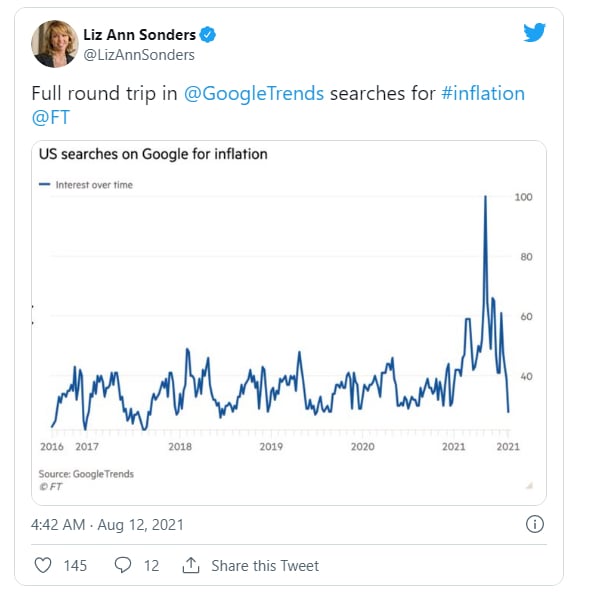Screenshot Description: The image is a screenshot featuring Liz Ann Sonders. At the top, her name "Liz Ann Sonders" is prominently displayed. Liz Ann Sonders has shoulder-length blonde hair and is wearing a black top complemented by a necklace. 

In the lower-right corner, the Twitter logo is visible, symbolizing that the original content might be related to a tweet. The text on the screenshot includes "Full round trip in @GoogleTrends" and "searches for #Inflation @FT," with the usernames and hashtags highlighted in blue, indicating clickable links.

The screenshot also contains a graph titled "U.S. Searches on Google for Inflation." The graph has a blue line representing the interest over time in inflation-related searches. The timeline starts in 2006 with interest levels near zero, then shows a dramatic spike reaching a peak of 100 around mid-2021, before declining to approximately 10.

The source of the data is noted as Google Trends. The timestamp on the image indicates it was captured at 4:42 AM on August 12, 2021.